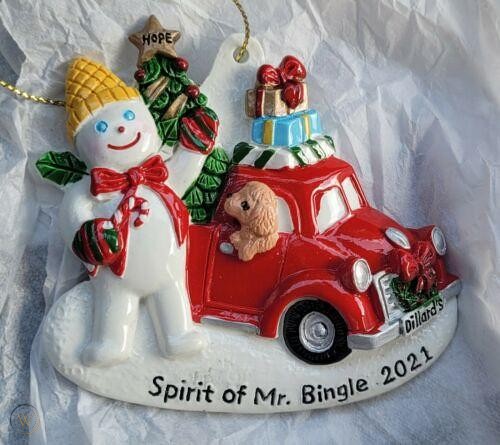In this image, we see a detailed, ceramic Christmas ornament laid on white tissue paper. The base of the ornament bears the inscription "Spirit of Mr. Bingle 2021" in black. The central figure is a cheerful snowman adorned with blue eyes, a red nose, and a red mouth. He wears a distinctive yellow hat resembling an upside-down ice cream cone, along with a red bow and multicolored mittens. One hand holds a candy cane while the other is raised in greeting. To his right, a bright red pickup truck is depicted with a light tan dog peeking out of the passenger window, gazing back at the snowman. The truck, detailed with a Christmas wreath on the front, stacks of presents on the roof, and black lettering that reads "Dillards," carries a decorated Christmas tree in its bed. The tree is adorned with red ornaments and a gold star that says "Hope" in black. The ornament is designed to hang, featuring a hole at the top through which a yellow twine loops, encircling the scene and anchoring it as a festive centerpiece.